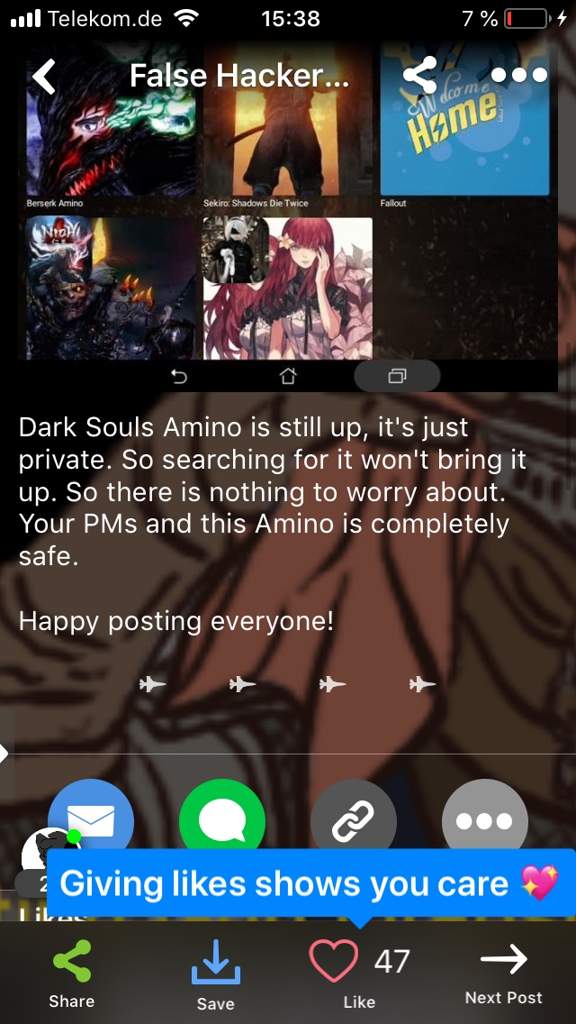The screenshot, captured at 15:38, displays a mobile phone screen with the telecom provider "telecom.de" indicated at the top. The battery level is critically low at 7%, highlighted by a prominent red bar. The screen features a collection of five game icons. The upper left icon is labeled "Berserk Amino," showcasing anime artwork. Adjacent to it is "Secure Shadows Die Twice," followed by "Fallout," which displays a blue square with the text "Welcome Home."

Beneath these, there's another game title that includes the word "Knight" and an anime-themed game to its right. In the text area below, a message reads: "Dark Souls Amino is still up. It's just private, so searching for it won't bring it up. There's nothing to worry about. Your PMs and this Amino are completely safe. Happy posting everyone."

The interface also includes four icons resembling fighter jets, along with buttons for email, speech bubble, link, and a menu marked by three dots. A section below invites user engagement with the text: "Giving likes shows you care," accompanied by a heart with gold sparkles. Further down are icons for sharing, saving, liking (with a count of 47), and navigating to the next post, each labeled accordingly as share, save, like, and next post.